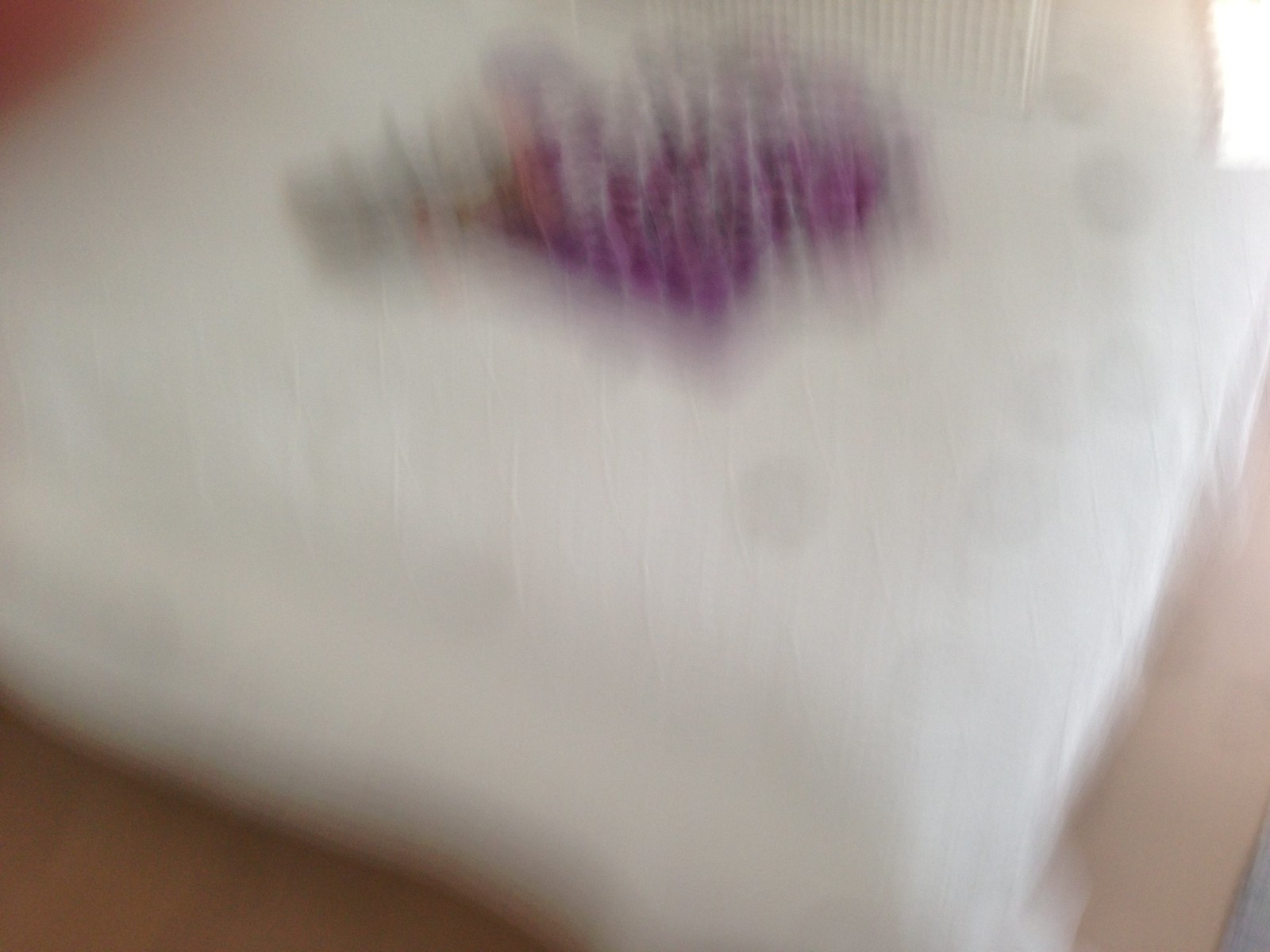This image is extremely blurry, dominated by a large white object with indistinct edges that appears to be situated on or surrounded by a brownish-beige surface, possibly resembling a table or a piece of wood. The center focus of the image seems to feature a white area interspersed with bubbles or circles, with hints of light gray. Accentuated by a mix of colors, the image shows a notable presence of purple and burgundy, perhaps in the form of embroidery or some other detail. The white area appears triangular, with a potential arrangement resembling an upside-down triangle. On the left side, subtle red tones can be observed, and towards the top middle, there is a square or checkered pattern in the background. Adding to the composition, the top right corner includes an area of white that might be light shining through or the presence of a window. The overall image is marked by its lack of definition, highly zoomed-in and shaky appearance, making it challenging to distinctly identify specific objects or features within the scene.